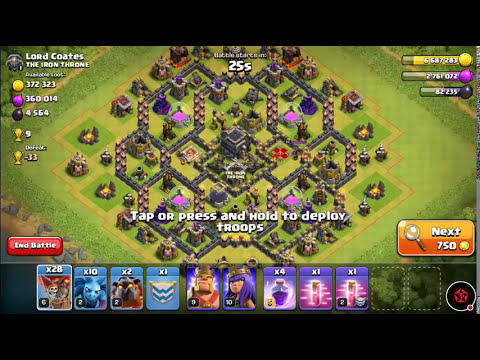This image is a screenshot of what appears to be a video game, possibly "Clash of Clans" or a similar world-building strategy game. The main view presents an aerial or diagonal perspective over a grid-patterned green meadow with various shades of green, brown, and yellow. Scattered across the scene are intricately arranged walls, buildings, and small castles, indicating a well-developed fortress.

At the top left of the screen, the text "Lord Coates, the Iron Throne" is displayed, accompanied by various numerical stats such as 372-323, 360, 014, and 4564, along with colored circles (yellow, purple, blue) likely representing different resources like gold or elixir. The top right corner features additional game information, including health or points indicators and an "End Battle" button in white text on yellow, gray, and brown backgrounds.

Prominently, mid-screen in white text, the instruction "Tap or press and hold to deploy troops" suggests active participation in troop management. At the bottom of the screen are nine rectangular icons resembling playing cards in a row, with numbers (e.g., x28, x10, x2) indicating the quantity of each troop or item available. There are 11 slots in total, with two outlined in dotted white lines, showing they are empty. Some cards feature characters or shields, and each has a star in the upper right corner.

On the bottom left, the "End Battle" button is present, and the bottom right includes a "Next 750" button with a magnifying glass icon, suggesting progression or currency cost. Additionally, various icons and avatars representing objects, food, soldiers, and gold line the bottom-most part of the screen, adding a layer of strategic options for the player.